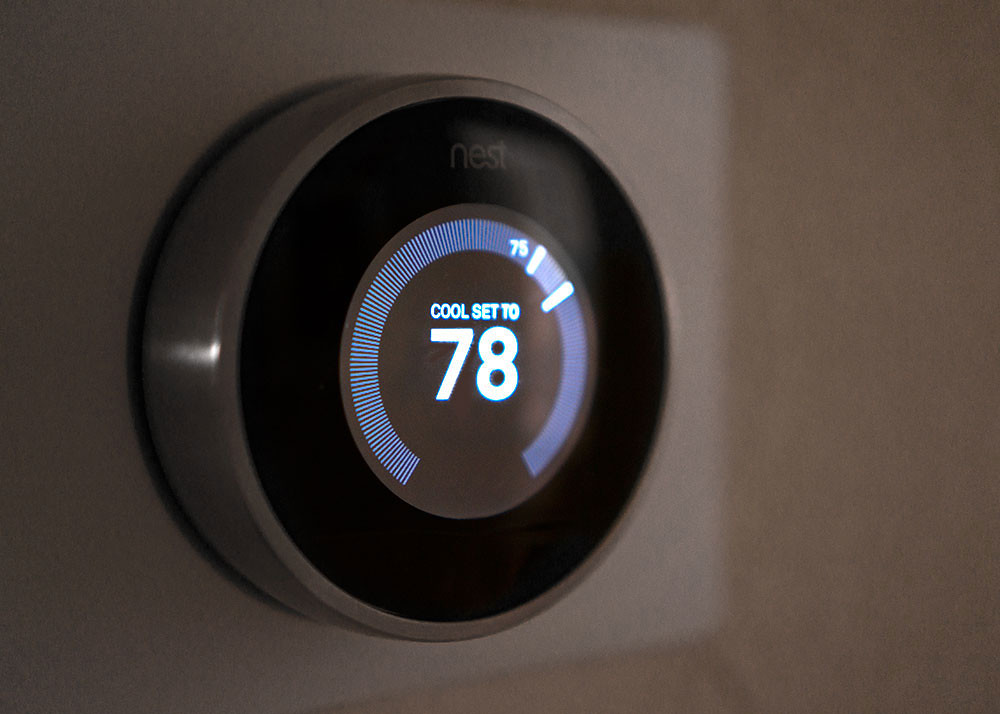This photograph captures a stylish and modern smart thermostat mounted on a wall, dimly lit to create a moody, shadow-infused atmosphere. The wall's color is indistinguishable due to the darkness, but it could be a neutral tone such as white or gray. The thermostat itself is circular, resembling a disc with a flat-edged rim approximately an inch and a half wide. Its design is reminiscent of a push-activated battery-powered light, featuring a sleek silver ring that encircles a black center.

In the middle of this black center, which resembles an eye, the brand name "Nest" is clearly visible at the top, displayed in lowercase letters that match the silver of the outer ring. The central "pupil" is illuminated, featuring a precise meter with lines encircling the iris-like display. Prominently displayed in the center of the thermostat is the text "Cool set to 78," indicating the current temperature setting. This stylish, modern device highlights both functionality and aesthetic appeal, making it a likely candidate for a product image.